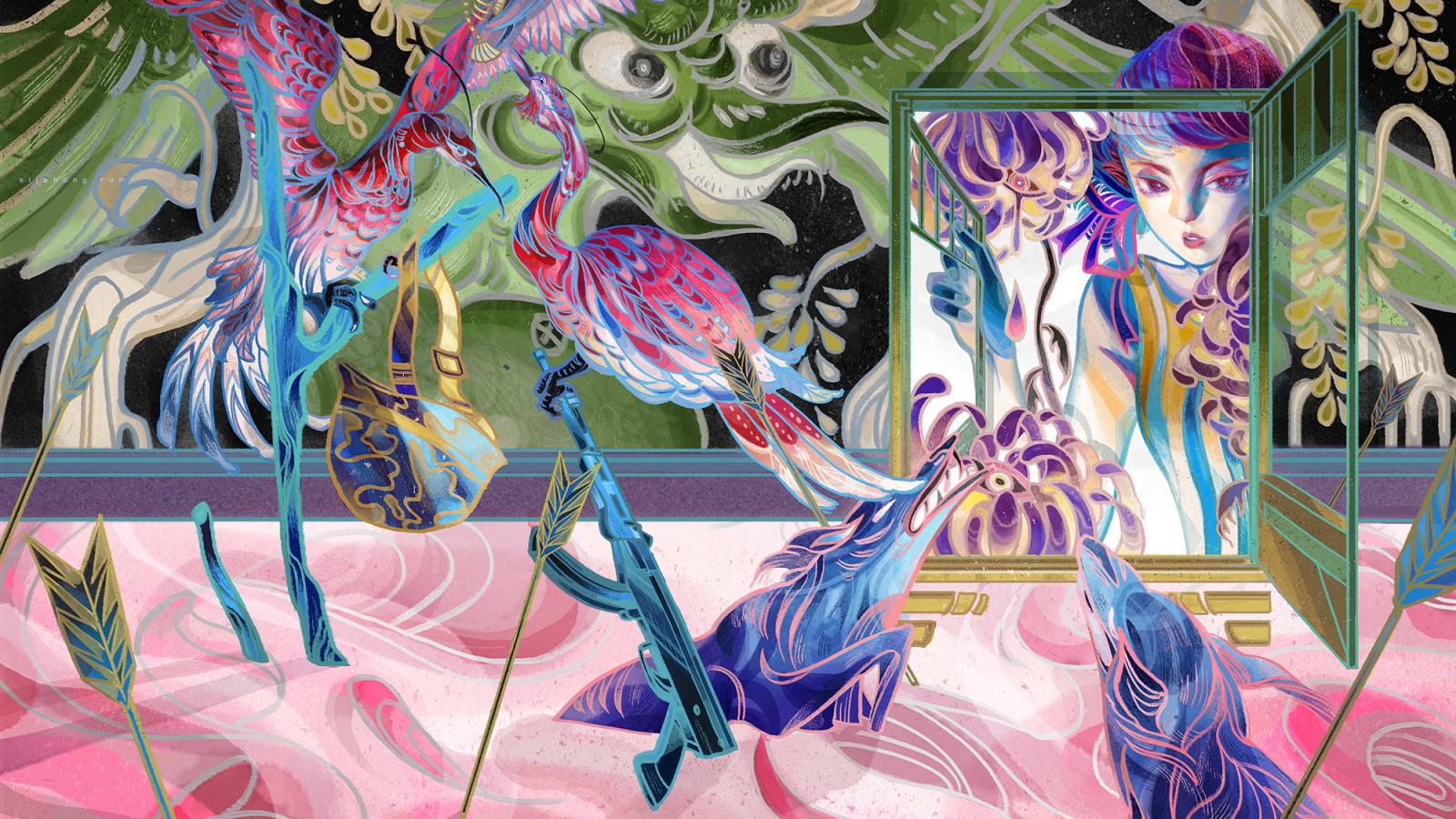This is an abstract and heavily stylized illustration teeming with a myriad of vibrant, pastel colors. Predominantly using shades like magenta pink, royal blue, pastel greens, and varying hues of purple, the scene is densely packed with various elements. 

The bottom third of the frame features a pink floor adorned with dark pink swirls, outlined in white. Emerging from this floor are two blue, dog-like creatures with sharp white teeth and pink outlines, angling upward from the center and bottom right. Scattered across the floor are arrows with blue interiors and golden outlines, alongside a teal blue assault rifle outlined in light blue, angling to the left. A purple baseboard marks the start of a black wall backdrop, against which a green, dragon-like figure with exaggerated features gazes to the right.

In the right part of the frame, an open window with a green and yellow frame emerges from the floor. Through this window, a person with pale yellow to purple skin, purple hair, and a yellow and blue striped shirt is visible. They are surrounded by purple flowers. Floating in front of the black wall is a blue branch with another branch extending to the right, supporting two pink birds with light blue outlines. One bird gazes downward at a soldier’s helmet, blue with golden squiggles, hanging from a rightmost branch. The other bird faces left, its talon clasped around the tip of the assault rifle barrel. The entire composition conveys a busy, eclectic tapestry of imagery, blending physical and digital artistic styles seamlessly.